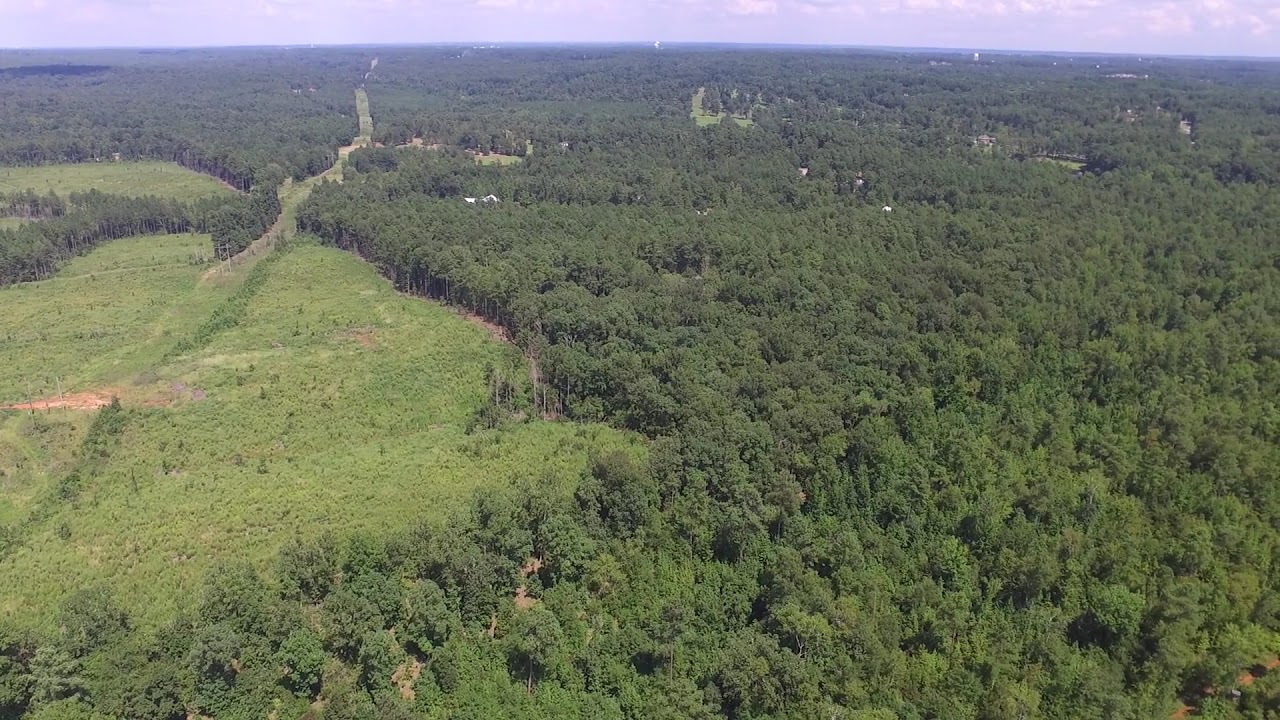This is an overhead aerial view of a vast and dense forest that occupies approximately 75% of the right side of the image, extending all the way to the background. The canopy is thick with tall, green trees, creating a lush, unbroken expanse of foliage. Along the top edge, a narrow band of sky is visible, tinged with a purplish hue and sporadically dotted with clouds. On the left side of the image, there is a noticeable cleared section that forms almost a triangular or rectangular patch. This area is significantly lighter in color, covered with green grass and sparsely populated with clumps of trees. A prominent path or road cuts through this cleared section, extending into the distance and possibly used for logging purposes given its cleared nature. There are no visible buildings or text in the image, emphasizing the natural, undisturbed essence of the landscape.